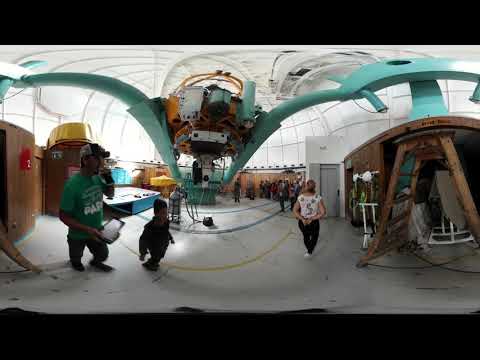The image captures a construction site with a subtly distorted perspective. In the foreground, from left to right, there's a man wearing a green shirt with "Poppy" written on it, and a hat, who appears to be eating something. His legs seem unusually short due to the image's curvature. Next, a small child in a black outfit and stocking cap is walking near him. Further to the right, a woman with long hair is walking away, dressed in black pants and a white shirt adorned with a flowered pattern that some described as having a dollar sign. A wooden ladder stands on the right-hand side of the image.

The setting features a white, semi-transparent ceiling, allowing sunlight to pass through, with green beams and pipes above. The ceiling also contains multiple compartments, possibly part of a central machine or structure with green arms, and yellow, gray, white, and black elements. The walls are a mix of white and brown wood, with a gray door in the back, possibly an elevator. Additional details include yellow and blue lines on the concrete floor, indicating future construction plans, and various white objects scattered in the background. The overall scene suggests an indoor setting, likely a school or similar building undergoing renovation or some sort of project work.